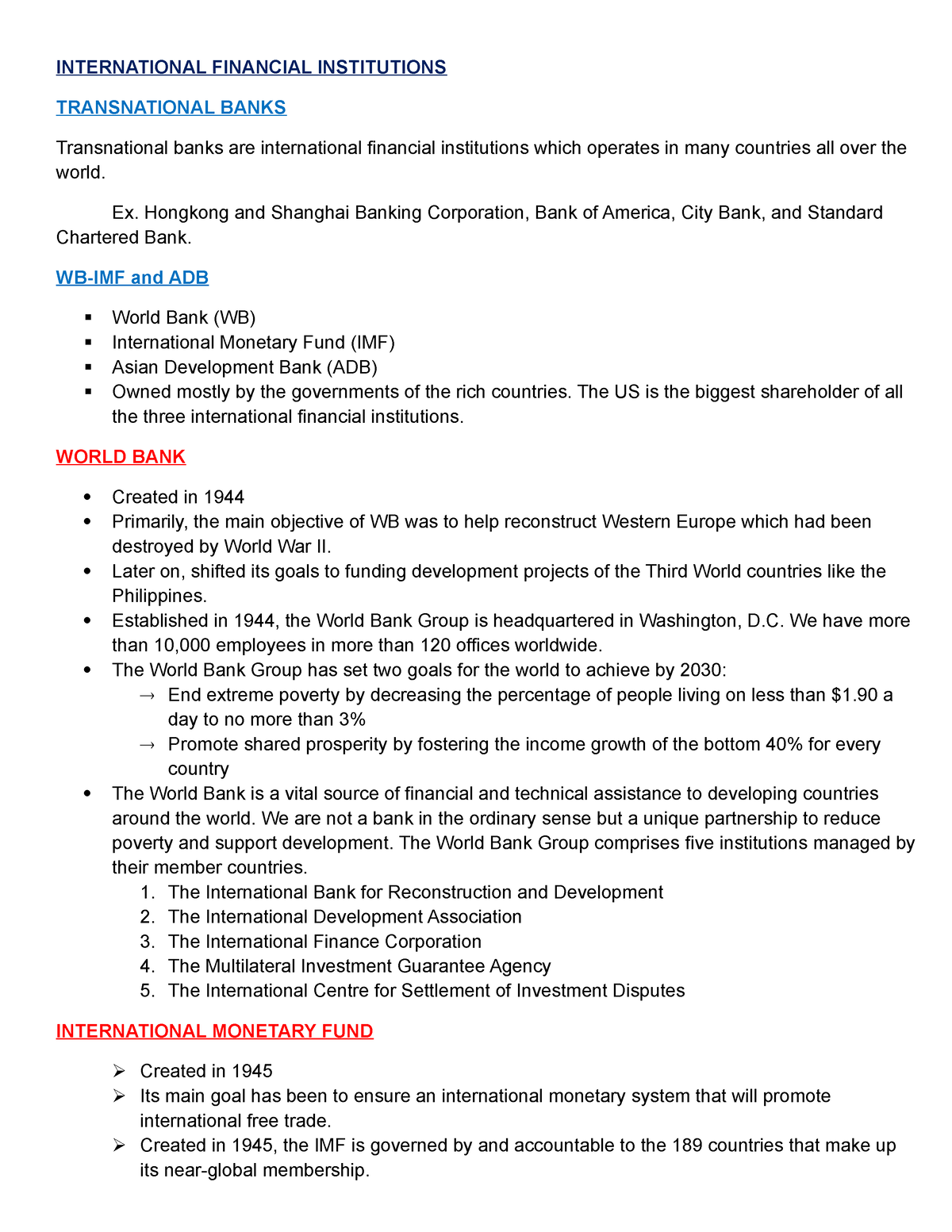This screen capture displays a detailed document on international financial institutions, focusing on entities like transnational banks, the World Bank, and the International Monetary Fund (IMF). The header "International Financial Institutions" is prominently typed, followed by a "Transnational Banks" subsection in blue text. This section defines transnational banks as those operating globally.

Further down, the document lists abbreviations WB-IMF and ADB in blue text, accompanied by four bulleted points elaborating on these banks. Below this section, "World Bank" is highlighted in red text and underlined, supplemented by six detailed bullet points discussing its history and mission. One point denotes the World Bank's establishment in 1944, followed by specific 2030 goals, such as eradicating extreme poverty by reducing the number of people living on less than $1.90 a day to 3% and promoting shared prosperity by increasing the income growth of the bottom 40% in every country.

At the bottom of the document, "International Monetary Fund" is mentioned, stating its creation year, 1945, adding context to its inception.